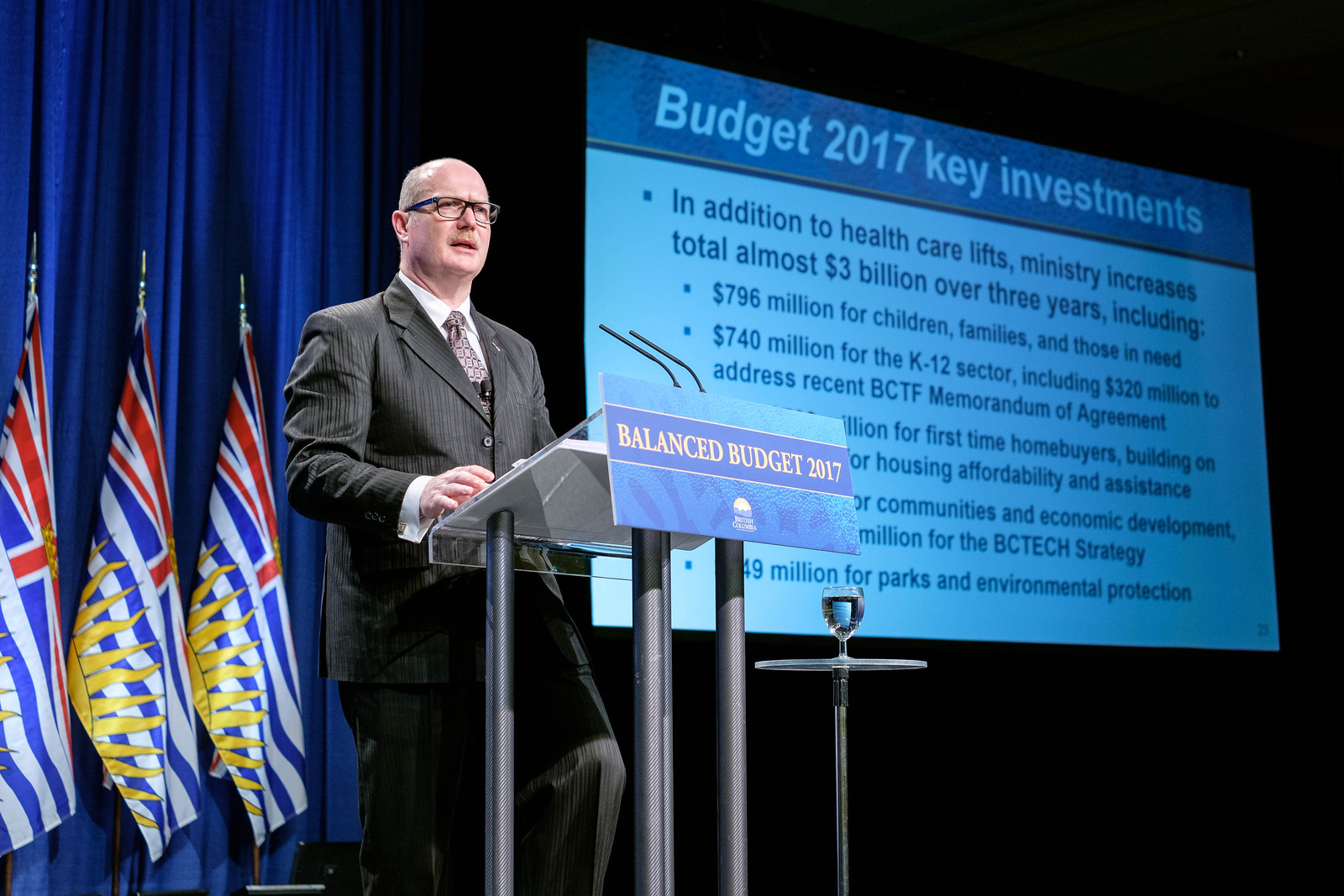The image depicts an older, bald man with glasses and a partial mustache, standing at a podium on a stage. He is wearing a gray suit, white shirt, and brown tie. The podium features a blue placard that reads "Balance Budget 2017." Next to him, a large projection screen displays a slide with the title "Budget 2017 Key Investments" in large white font on a dark blue banner. The slide details budget allocations, including significant investments in health care and education, but much of the text is obscured by the podium. The stage is draped with blue curtains and adorned with three flags that are red, white, and blue with stripes, bearing a yellow sun logo. Additionally, there is a table with a glass of water to the man’s side.